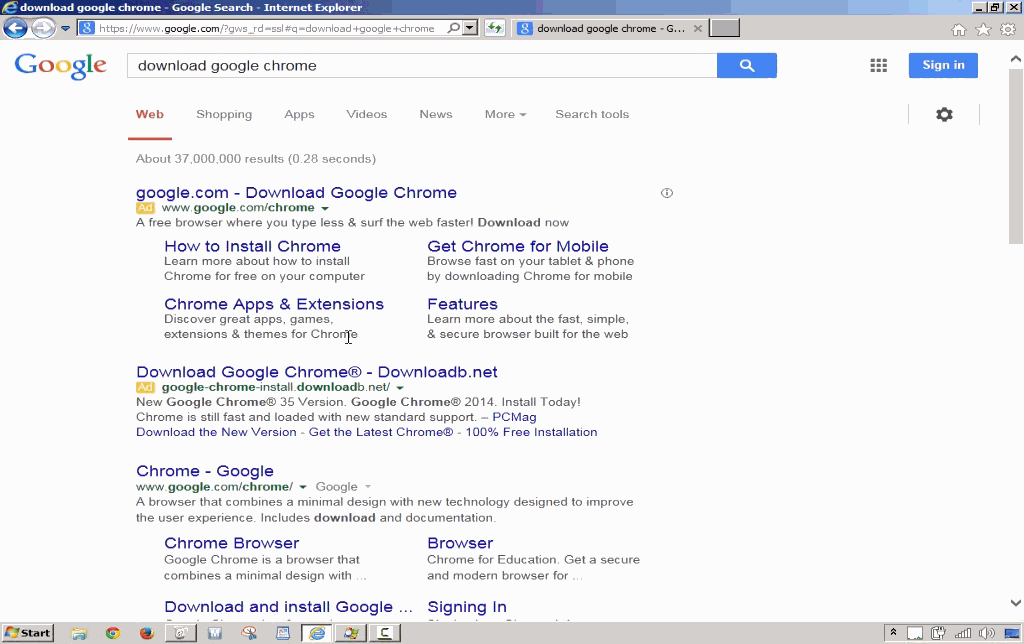A detailed and cleaned-up caption for the image could be:

"This screenshot captures a desktop screen running Internet Explorer, easily identified by the iconic 'E' logo in the upper left-hand corner, signifying an older version of the browser. The user is on the Google search results page, having typed 'download Google Chrome' into the search bar. This search query is also reflected in the browser's title bar, which reads 'Download Google Chrome - Google Search - Internet Explorer.'

In the upper right of the browser window, standard control icons for minimizing, restoring, and closing the window are visible. Below these, there are icons for home, favorites, and settings. The Google search page displays a 'Sign In' button on the right-hand side and offers various search options including Web, Shopping, Apps, Videos, News, More, and Search Tools.

In the bottom right-hand corner of the screen, several system icons are visible: a star, an unknown white rectangle, a battery or charger status icon, a fully connected Wi-Fi signal icon, a speaker icon, and a Windows wallpaper indicator. The taskbar also denotes that the user has four tabs open in the browser.

Overall, this screenshot illustrates a user attempting to download Google Chrome via an outdated version of Internet Explorer, revealing a blend of legacy and modern elements on their desktop."